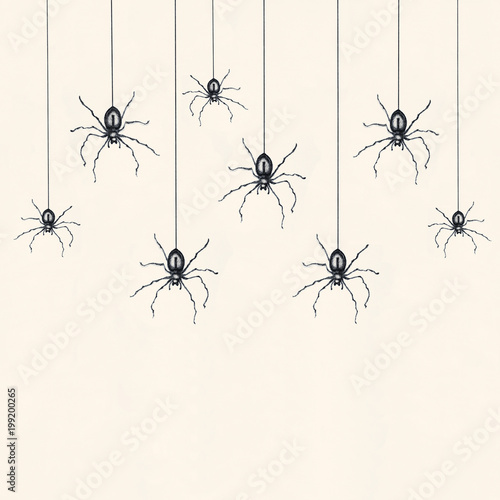This image is a square format, black line art illustration featuring eight spiders descending from the top on single threads of black webbing. Each spider has a black and gray abdomen, shiny bodies, and eight scraggly, wiggly legs. The spiders vary slightly in size and are positioned at different heights, with the lowest ones reaching about two-thirds down the image. The background is a very light tan or cream color. A prominent watermark reads "Adobe Stock" diagonally across the image, and in the bottom left corner, the text "Adobe Stock number 192-00265" is written vertically. The overall style is simple clip art with a clean, minimalistic design.